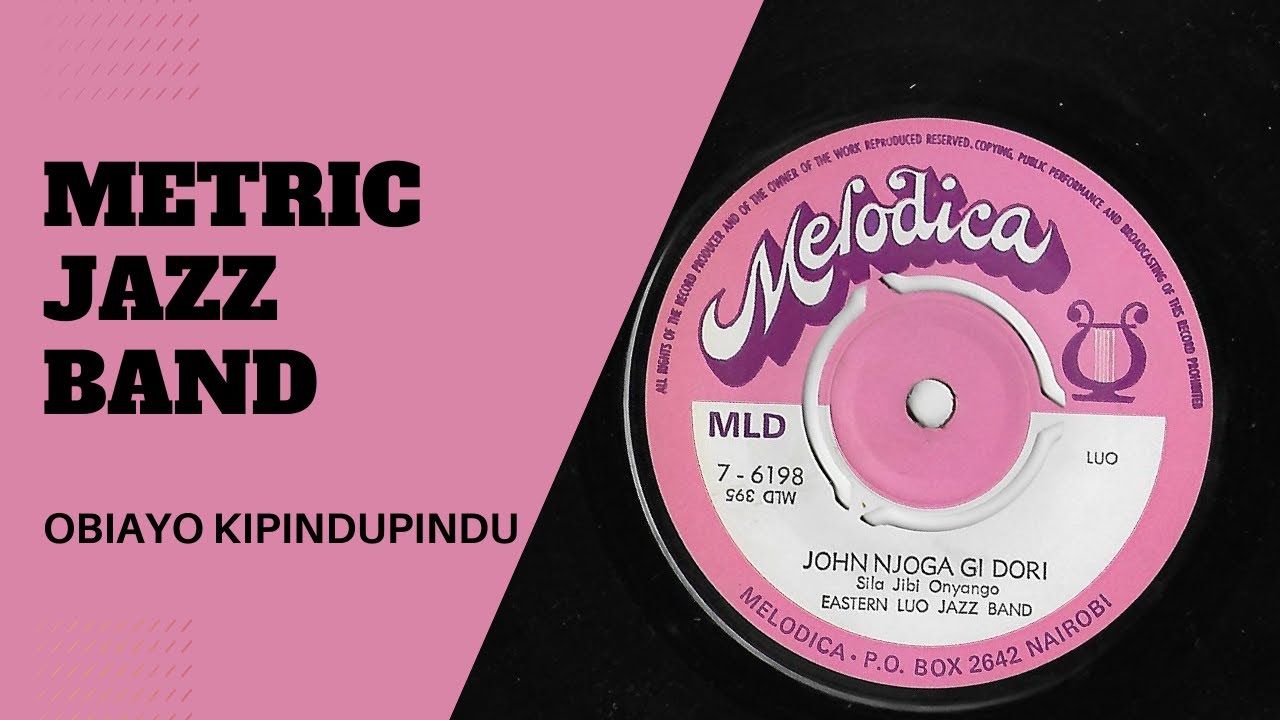The image displays a business card with a diagonal divide; the left half is pink with black lettering, and the right half is black, resembling the center of a 45 single record. On the pink side, the card reads "Metric Jazz Band" followed by the name "OBIAYO KIPINDU." The black side mimics a record label and features the text "Melodica" in pink with a small harp image. Additional information includes “John Njogadjiduri,” “Sela Gbon Yongo,” “Eastern Luau Jazz Band,” catalog numbers "MLD 7-6198" and "MLD 395" (printed upside down), and the contact information “Melodica, P.O. Box 2642, Nairobi.” The record label design has pink, white, and purple accents, and includes a half-circle graphic along with a disclaimer about the rights of reproduction and performance.